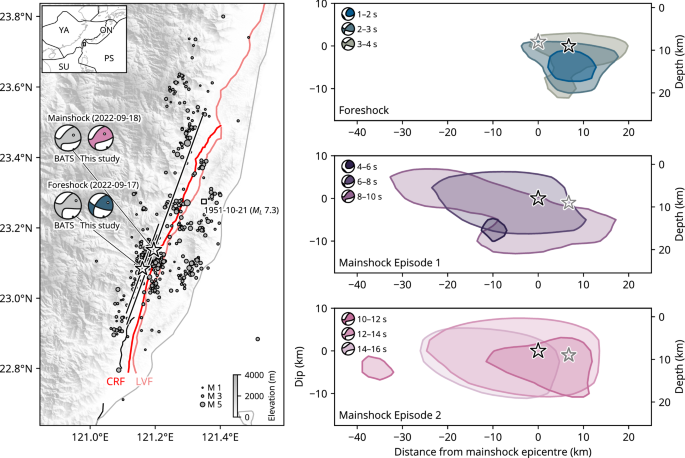The image is a detailed diagram featuring a series of graphs and maps, likely related to earthquake monitoring or seismographic data. On the left, there's a large rectangular map of a landmass, spanning from 28.8 to 22.8 degrees north latitude and from 121.0 to 121.4 degrees east longitude. The map, primarily in gray and white, is dotted with numerous black circles and stars, and features a prominent red line that stretches diagonally across. Key annotations include "1951-10.21M7.3" and "Mengshak 2022-918". The map includes a legend at the bottom right indicating elevation in meters and various markers "M1, M3, M5".

Adjacent to the map, the right side of the image contains three vertically stacked panels, each labeled: "Foreshock", "Mainshock Episode", and "Mainshock Episode 2". These panels function as accompanying charts, illustrating data with vertical and horizontal axes marked in kilometers and seconds respectively. The top panel features blue graphical elements, the middle panel uses purple hues, and the bottom one is adorned with pink shapes. These panels depict data with depth and distance measurements, and each includes stars and distinctive colored shapes that convey specific events or data points related to the seismic activity being studied.